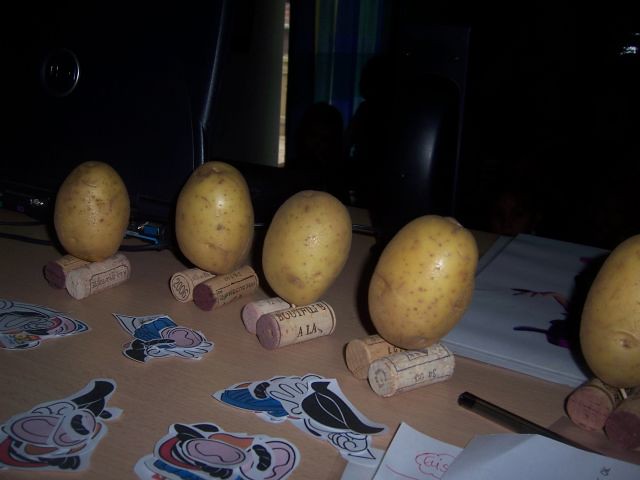In this detailed photograph, the focal point consists of five large, raw russet potatoes, possibly white potatoes, each balanced atop two sideways wine bottle corks, amounting to a total of ten corks. These potatoes, unpeeled and with their golden skins intact, are positioned upright on the corks, creating a curious and somewhat surreal scene. This setup is on a brown-topped desk or table. In front of the potatoes and corks are several small stickers, some representing cartoon body parts, suggestive of Mr. Potato Head accessories. Also visible on the table are other piles of stickers of various cartoon characters, miscellaneous pieces of paper, a drawing pen, and a very dark curtain serving as a backdrop.